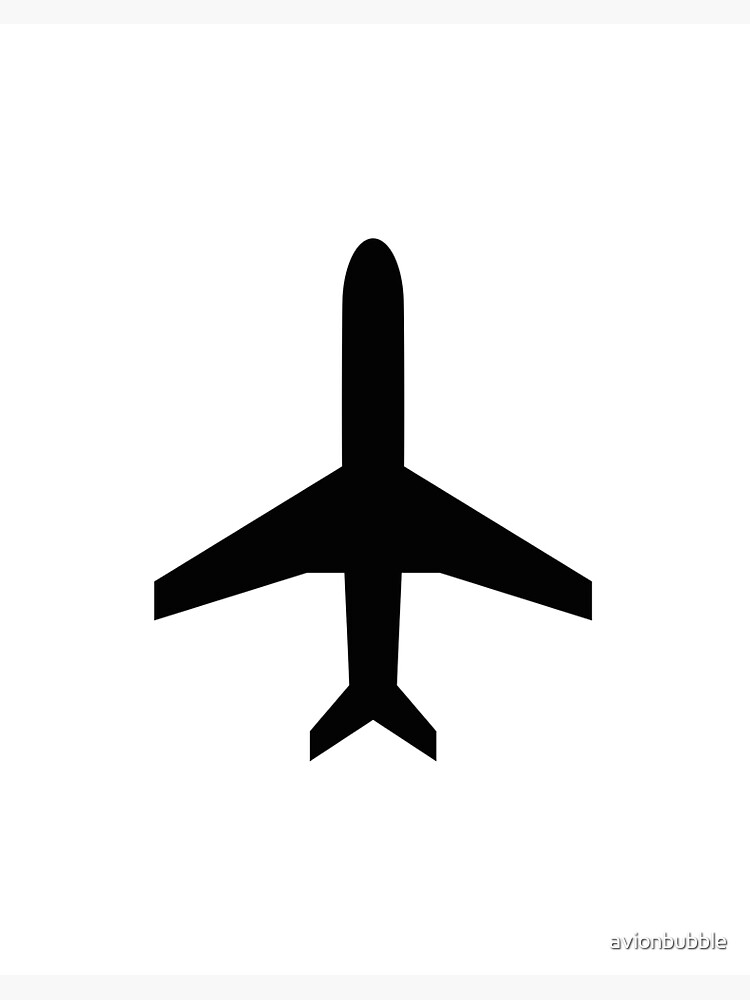The image features a stark, minimalist black and white design. Central in the composition is a black silhouette of an airplane, viewed from a bird's-eye perspective against a pure white background. The plane, entirely black and symmetrically depicted, includes distinguishable wings jutting out from the middle and a V-shaped tail. Its direction appears to be ascending. Down in the lower right-hand corner, the image includes the text "Avion Bubble" in lowercase letters, with a slight shadow effect, possibly suggesting a logo. The simplicity and clarity of the design, resembling an airport symbol or a figure in a commercial aviation manual, emphasize the black airplane as the sole focus, making the image straightforward and easy to interpret.